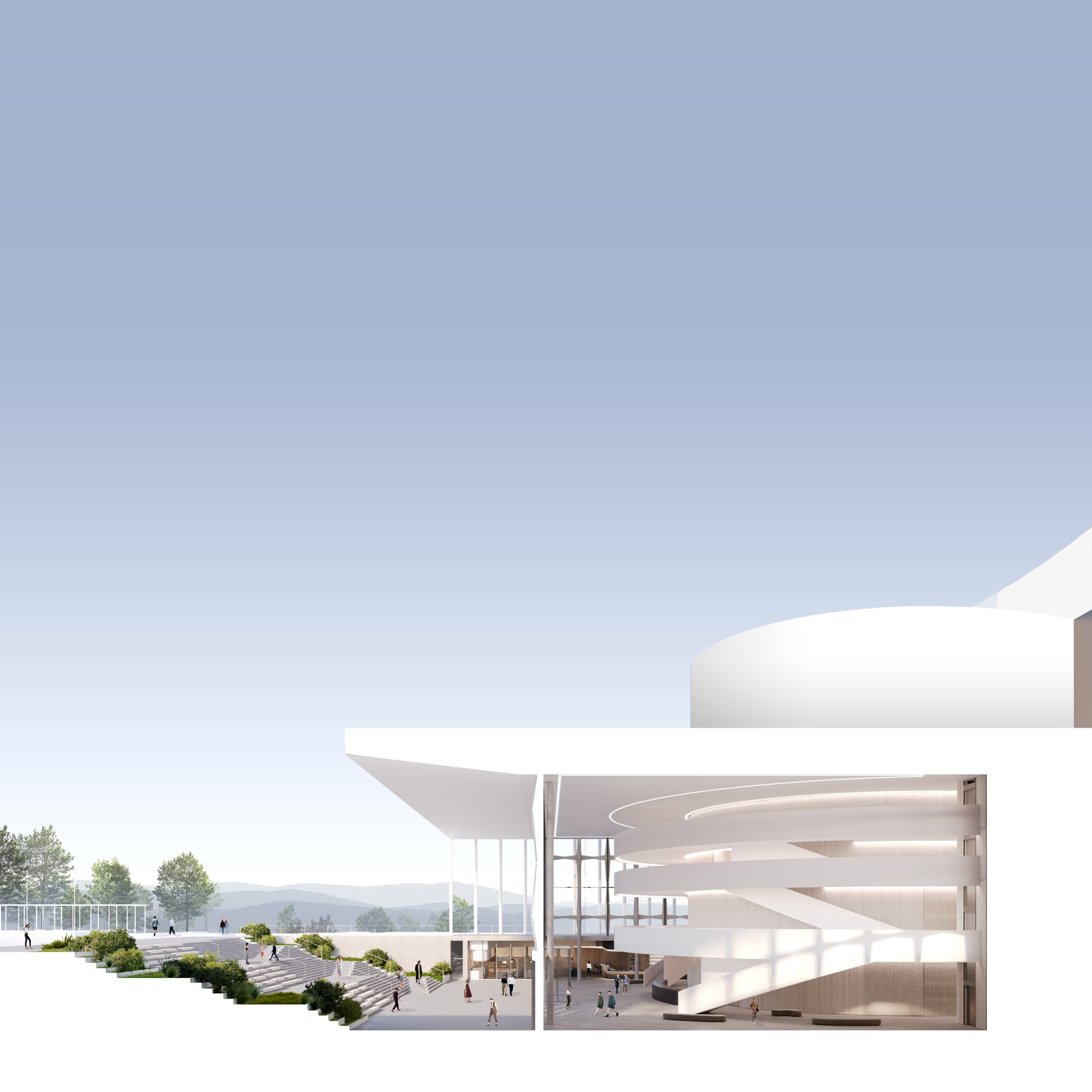This detailed and highly realistic artist's rendition, likely created using computer-generated 3D art, presents a striking profile shot of an enormous, ornate white building against a perfectly blue sky. The building, reminiscent of a modern museum with a grand and futuristic design, is characterized by its immense size and standout features. It occupies approximately half of the image, with the other half dominated by an expansive, empty sky.

The structure incorporates a circular design with a prominent spiral staircase ascending through different floors, suggesting a continuous internal pathway. The uppermost part of the building showcases a distinct rounded, bowl-like roof. The front facade features three grand flights of stairs that rise from a granite courtyard at the base to an elevated entryway. Each side of the staircase is flanked by meticulously maintained green hedges and grass.

Moreover, the ground level, paved in white granite, is populated by numerous tiny figures of people, underscoring the building's monumental scale. In the far background, beyond the architectural marvel, there are hints of water bodies and lush trees, adding depth and context to the setting. The entire scene is illuminated by a combination of natural and artificial white lighting, enhancing the pristine and majestic appearance of the structure.